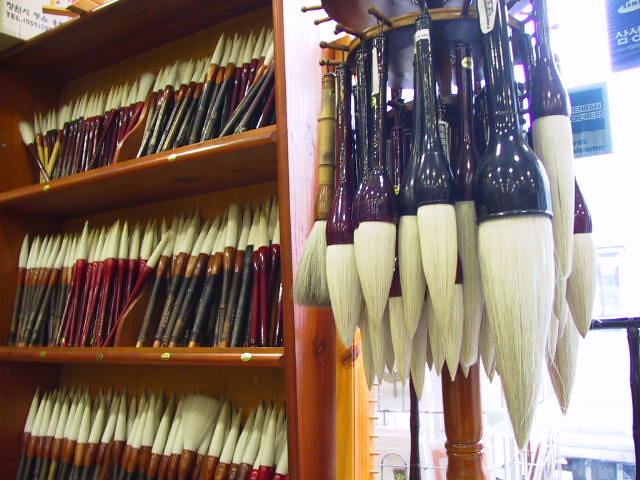This photograph captures the brush section of an arts and crafts store, featuring a variety of brushes primarily used for calligraphy, ink drawing, or large arts and crafts projects. The scene showcases a well-lit display area with a bookcase on the left that holds an extensive collection of brushes, each coming to a fine point, arranged with the handles at the bottom and the bristled ends at the top. The bookcase, which has three visible shelves, displays brushes with dark, shiny brown handles, some of which are maroon. The top shelf holds smaller brushes, the middle shelf features medium-sized brushes, and the bottom shelf displays larger brushes. Many brushes have long, pointed bristles, varying in length from a few inches to almost ten inches, and some are described as being made from horsehair or other fine animal hair, suggesting their craftsmanship and potential high cost.

To the right, there is a round display where brushes are hanging upside down, showcasing their varying sizes and bristle lengths. The brushes on this turner have high-gloss purple handles, adding to the aesthetic diversity of the collection. In the background, a window illuminated by natural light is visible and features a sign indicating that American Express is accepted, alongside other advertisements that are not legible due to the image quality. The scene is rich in detail, with the diverse array of brushes organized in a manner that highlights both their artistic utility and visual appeal.